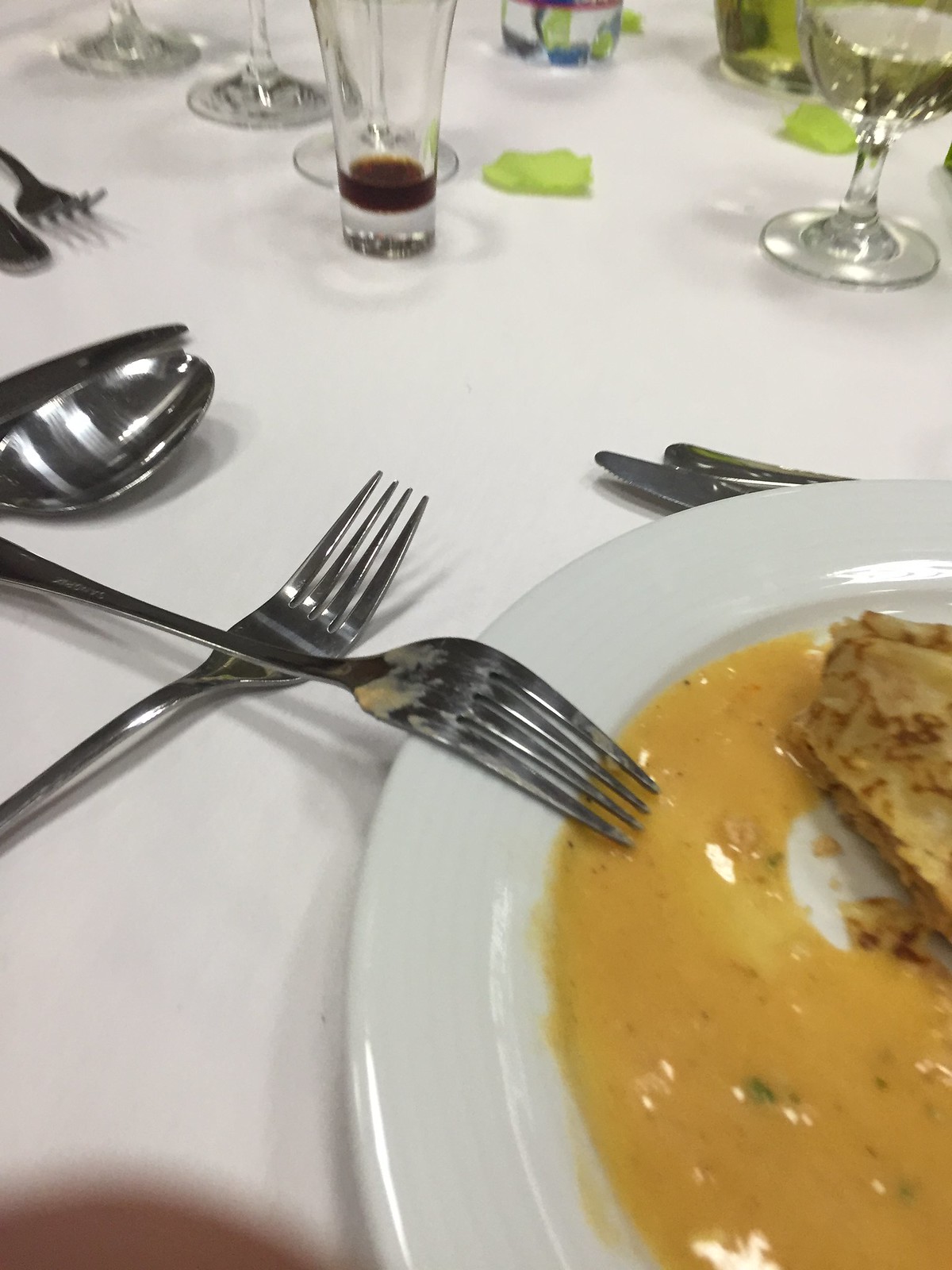This photograph captures a detailed scene of a banquet table adorned with a pristine white tablecloth. Positioned in the bottom right corner is a white plate featuring a piece of food, possibly chicken, surrounded by a light-colored gravy or sauce. An inverted, used fork with remnants of food rests on the edge of the plate. Above and to the side of the plate, a variety of meticulously arranged silverware, including additional forks, a spoon, a butter knife, and another fork, can be observed. A small glass, partially filled with a brown liquid, is also present on the table. Adding a touch of elegance, a floral centerpiece with delicate petals is displayed, along with some green paper leaves near the wineglass base.